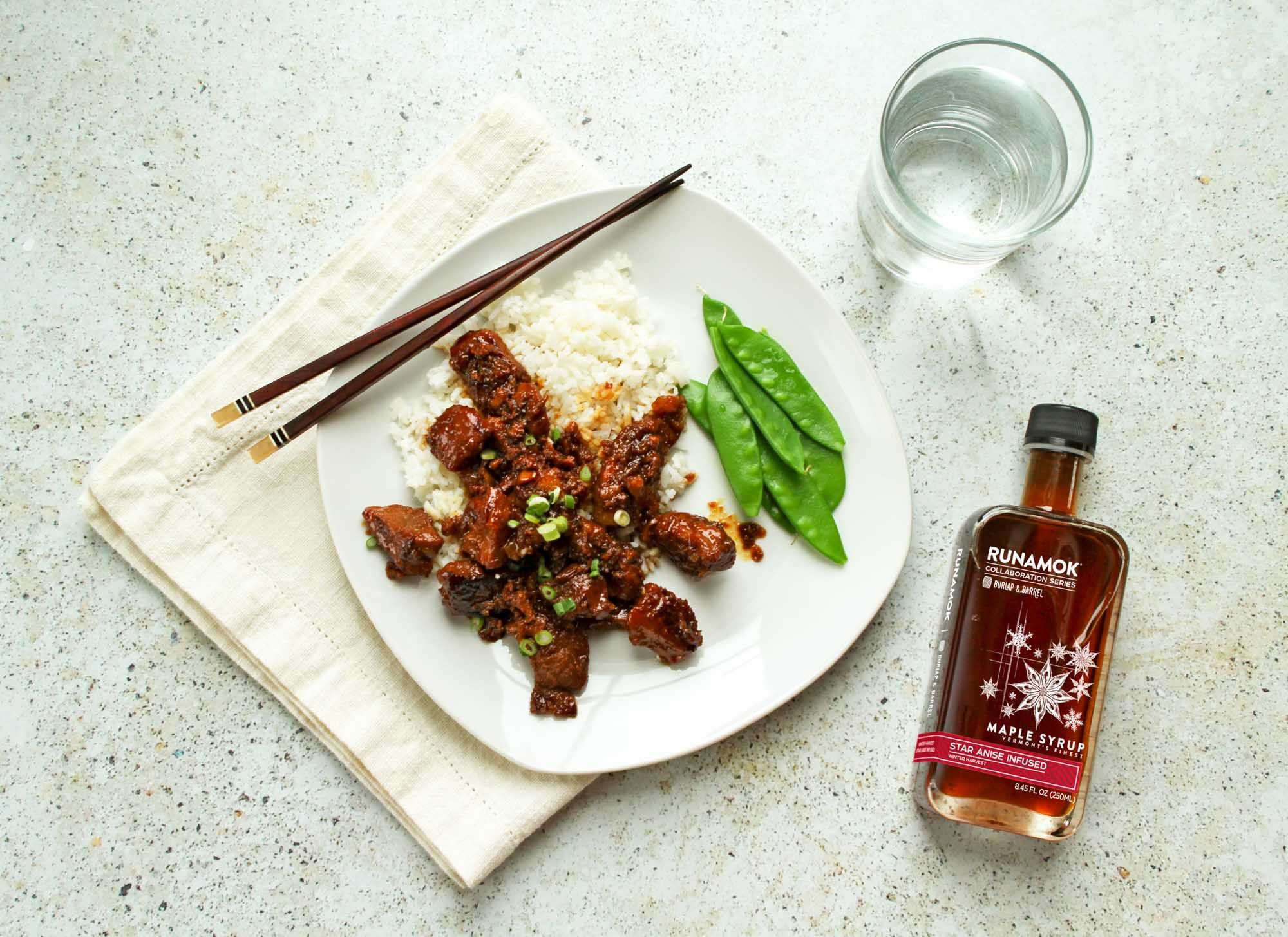The image showcases a meticulously plated dish of stir-fried meat in a red chili sauce, garnished with finely sliced scallions, all resting on a bed of pristine white rice. The meal is complemented by fresh, vibrant green snow peas arranged on the right diagonal of the plate. This culinary presentation is set on a white, square plate placed upon an ivory-colored cloth napkin. The entire setup resides on an elegant, faux marble countertop speckled with mica and silica, emulating a quartz surface. On the top left side of the plate, a pair of wooden chopsticks are neatly crossed, ready for use. Accompanying the dish, there is a glass of clear liquid—either water or vodka—positioned on the upper right side of the plate. Additionally, a bottle of Runamok maple syrup, adorned with white star-like designs, lies horizontally in the lower right corner, suggesting a unique infusion of flavors intended to enhance the stir-fried meat.